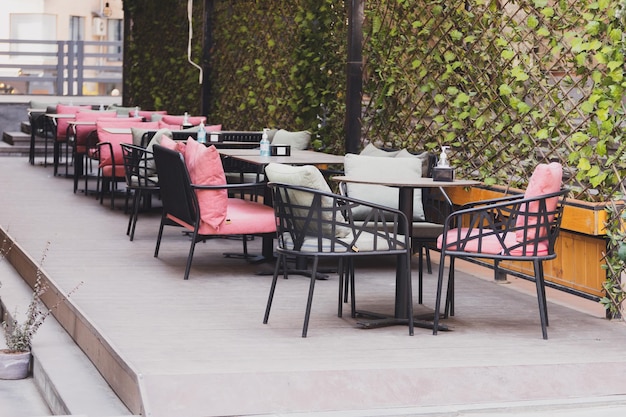This horizontal rectangular photograph captures an outdoor seating area on a restaurant or bar patio, possibly set on a rooftop in a city. The scene features a lineup of tables on a raised platform accessible by a couple of steps. There are four to five tables, with pedestals supporting either round or square tabletops. At each table, there are three to five gray metal chairs, many adorned with padded cushions in either light pink or gray cloth, some of which feature a geometric pattern. 

In addition to individual chairs, a few tables also have benches. The tables are uniformly equipped with a box of napkins and a small hand sanitizer bottle. Surrounding the seating area, there is a wooden backdrop and a lattice fence interwoven with ivy plants growing out of wooden planters. Visible towards the back left of the image is a railing and the windows of another building, reinforcing the elevated nature of the space. Additionally, there's a hint of umbrellas overhead, indicated by visible handles used to open or close them, providing shade on this urban oasis.